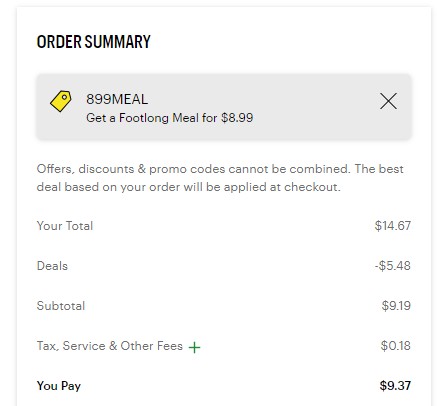This is a detailed screenshot of an order summary box from Subway. The top left corner prominently displays the title “ORDER SUMMARY” in uppercase black letters. Just below the title, there is a gray rectangular bubble featuring a yellow tag labeled “$8.99.” Adjacent to the yellow tag, the text reads “$8.99 meal.” Directly beneath this line, it offers a promotion: “Get a foot-long meal for $8.99.” On the right side of this gray box, there is an 'X' icon for closing the box.

Below the promotional offer, the message states: “Offers, discounts, and promo codes cannot be combined. The best deal based on your order will be applied at checkout.” Highlighting the financial details, the total initially is $14.67. However, deals amounting to $5.48 are subtracted, reducing the subtotal to $9.19. An additional tax of 18 cents brings the final payable amount to $9.37.

The background color of the box is white. Next to the "FEES" line, there is a green plus sign indicating additional details. The total dollar amount is bolded in black for emphasis. The entire document features a clean, simple design with clear, readable fonts to ensure an easy viewing experience.